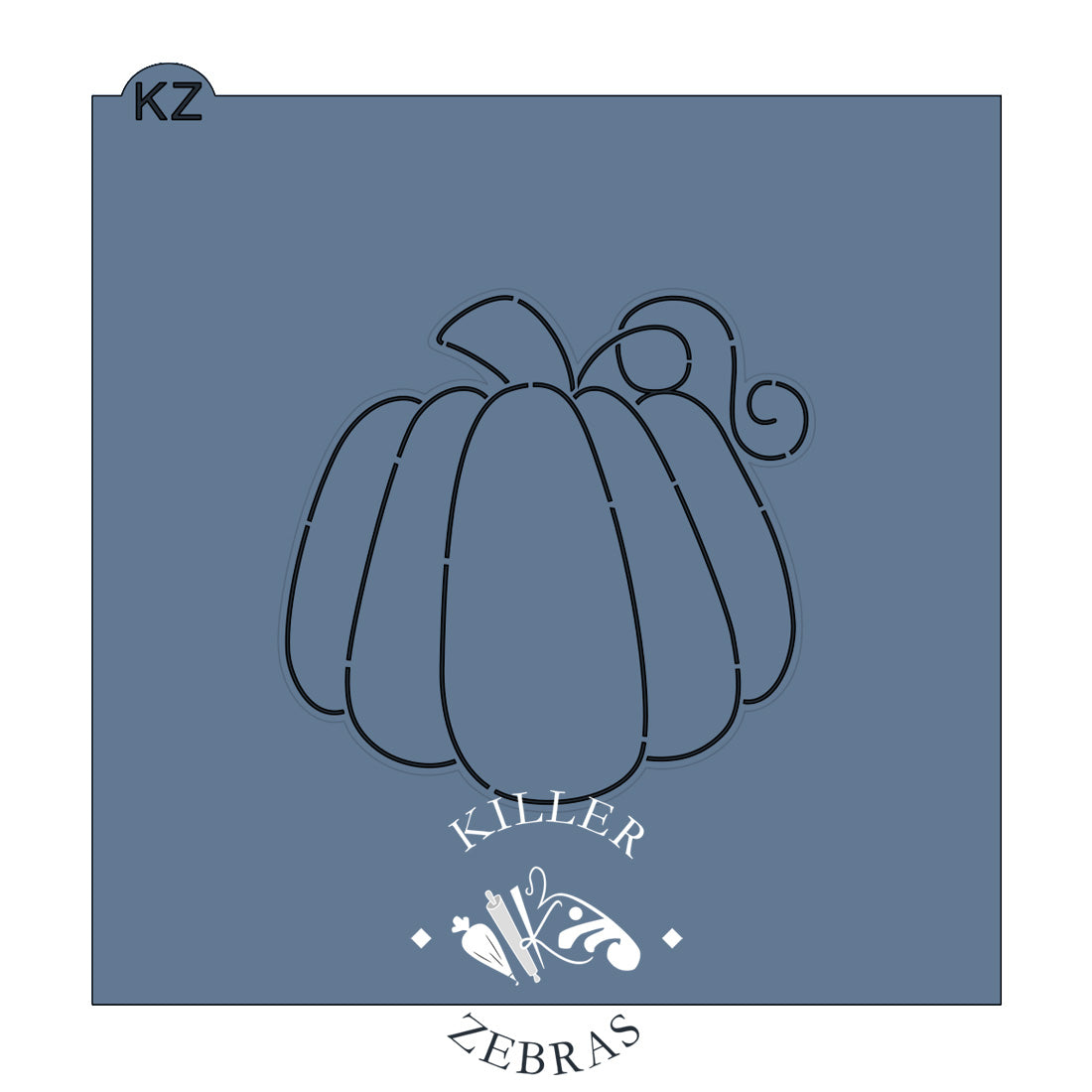This image features a detailed black sketch set against a light blue square background. Dominating the center is the outline of a pumpkin, clearly defined with all its characteristic grooves and a prominent stem at the top. Near the stem, a squiggly black line winds around, adding an extra flourish. Surrounding the pumpkin outline are various white sketches of fruits, including an identifiable carrot, arranged in a seemingly haphazard but intentional manner. Notably, in the upper left corner, there is a small, distinct bump containing the initials "KZ" in black. Below the central pumpkin sketch, the phrase "KILLER ZEBRAS" is prominently displayed in white letters. The ensemble of drawings and letters appears to convey a stylized logo or emblem, representing "KILLER ZEBRAS," and crafted with intricate attention to detail amidst the vibrant blue backdrop.